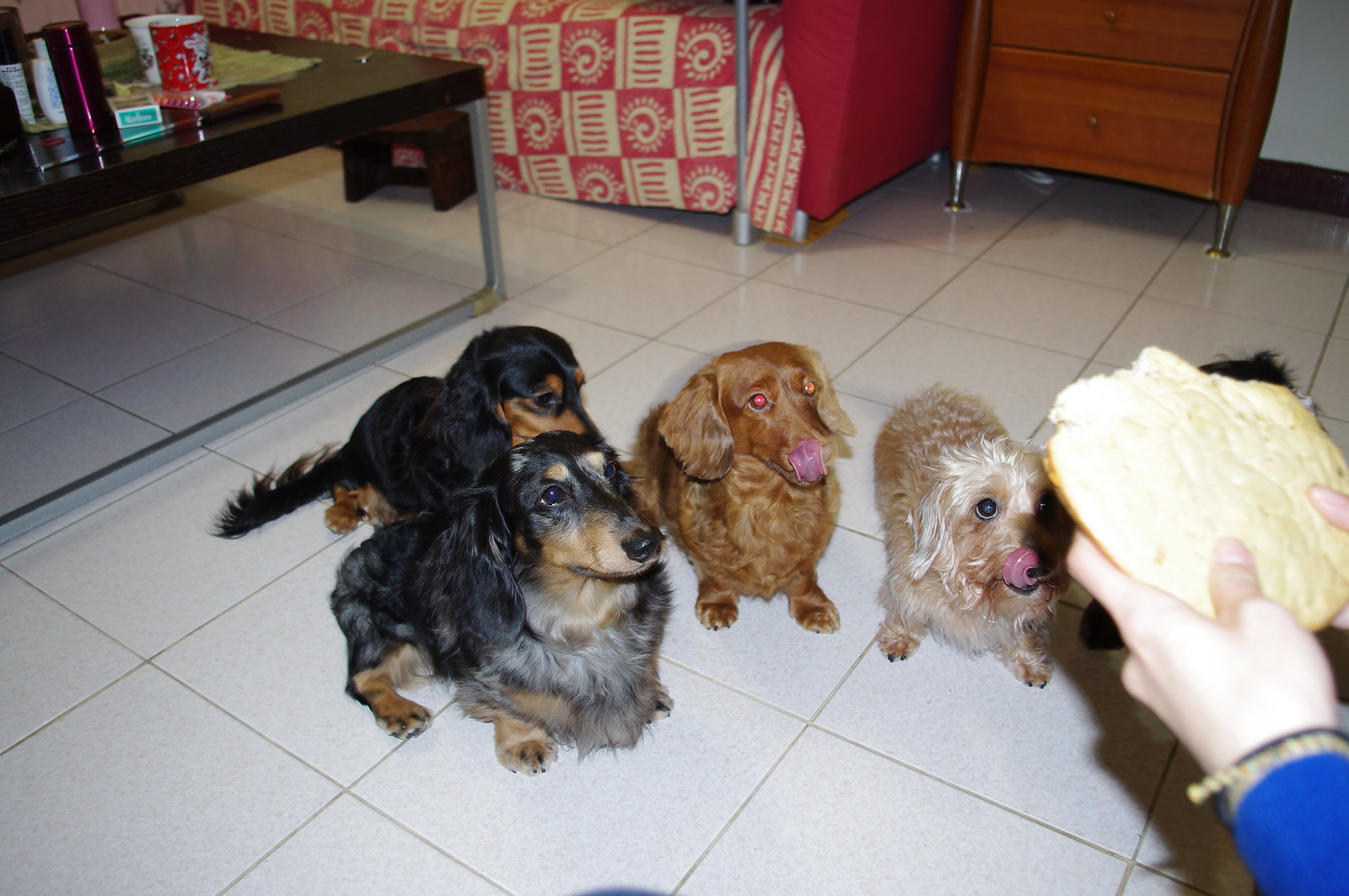The image depicts a cozy living room scene with five small dogs eagerly gathered in a semi-circle on a beige tile floor, their attention riveted on a piece of bread held by a person wearing a blue long-sleeved shirt and bracelets. The dogs, which include a mix of dachshunds and poodle-like breeds, display a range of colors: two are black and brown, with one featuring a gray chest, another is pure brown, and the last is light brown with curly fur. Two of the dogs, the brown and light brown curly-haired ones, are licking their lips in anticipation. In the background, the room is furnished with a red couch partially covered by a red and white blanket, a black metal coffee table, and a brown side table with two drawers, creating a warm and inviting atmosphere. The flash from the camera has illuminated the dogs' eyes, adding a lively sparkle to their eager expressions.